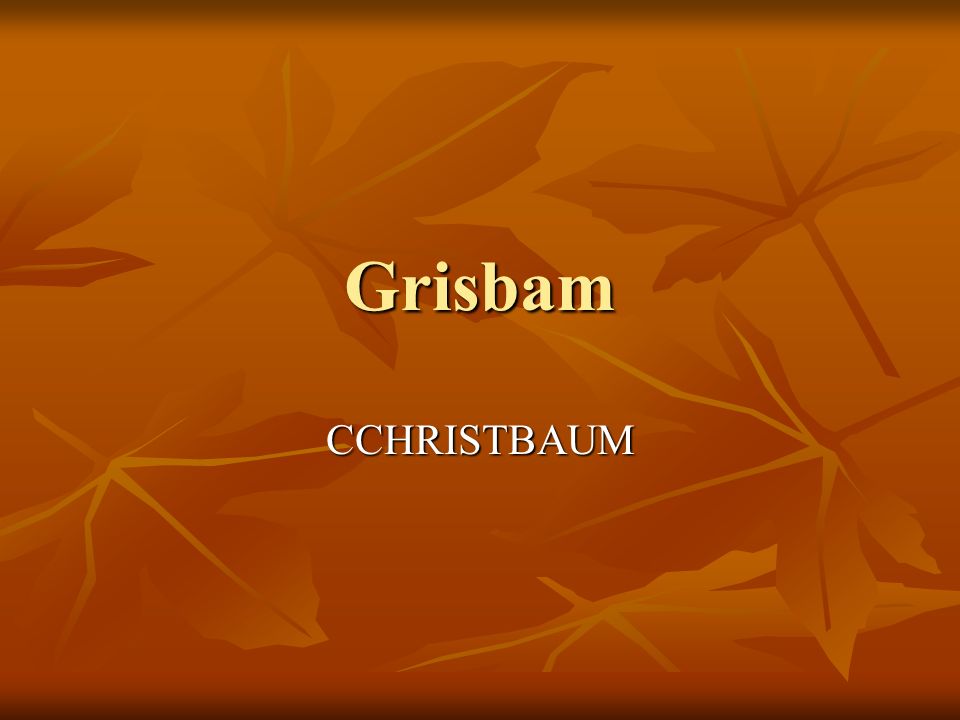The image, a computer graphic styled like a presentation slide or poster, features a rectangular design with an orangey-brown background that transitions from a darker shade at the top and bottom into a vivid orange. The background is adorned with tri-lobed leaf shapes, resembling maple leaves, in a slightly darker orange hue with intricate white and black veins. Centered in the graphic is the text, with the word "GRISBAM" in prominent yellow letters, shadowed to create depth. Directly beneath this, in white block capital letters, is "CCHRISTBAUM," also with a shadow effect. The overall aesthetic combines a gradient of orange tones and emphasizes the contrasting text and decorative leaf patterns.